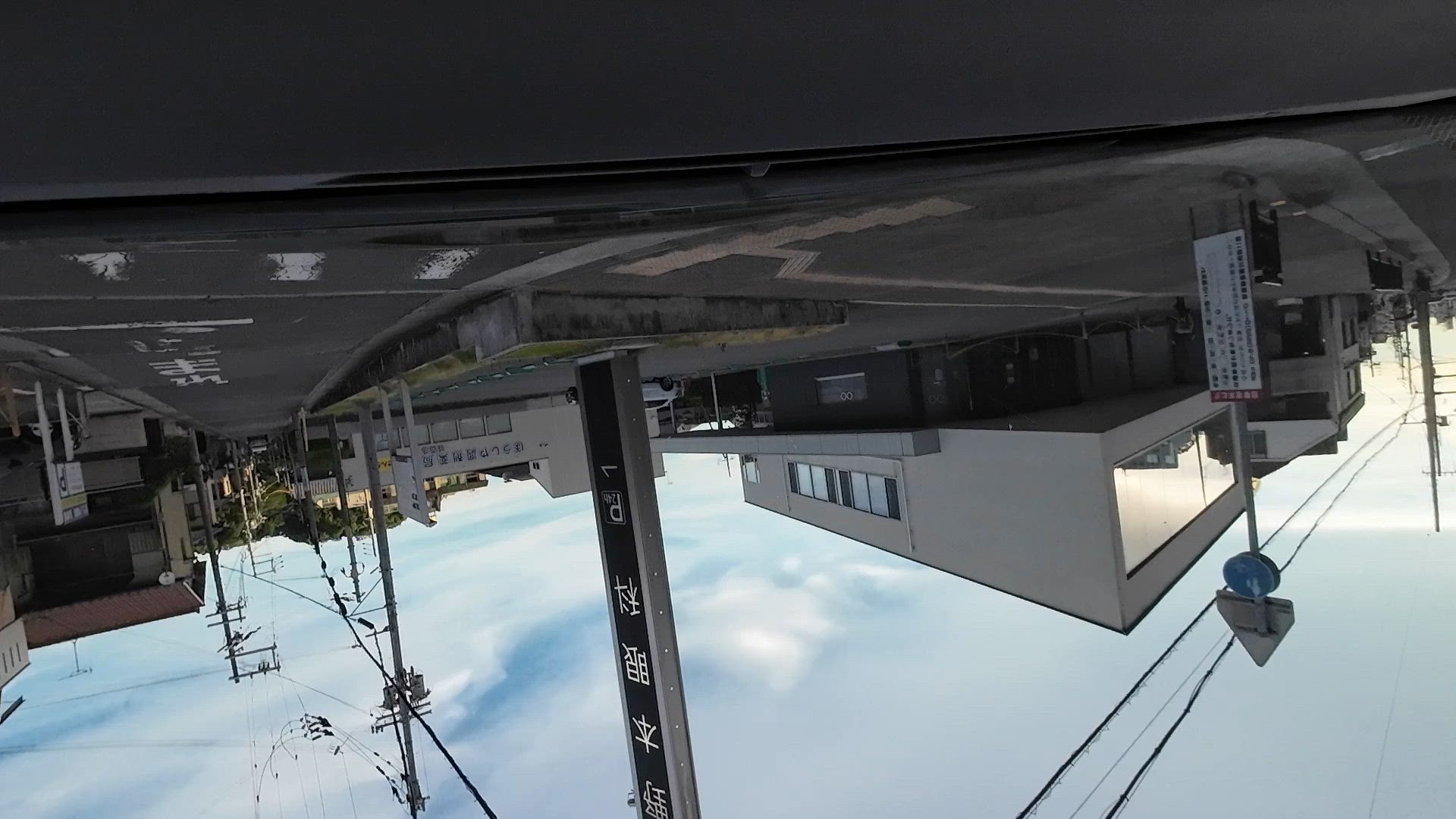The image is an upside-down photograph of a town or industrial area in an Eastern country, likely China or Japan, inferred from the presence of kanji characters on central signs. The perspective of the image means the road appears at the top while the sky is at the bottom. The predominantly clouded sky has a bluish-gray hue, suggesting an overcast day nearing evening. There are various buildings, including a white building with large windows on one side facing the street. The left side of the image features another structure with writing on it, surrounded by trees and possibly a house in the background. Power poles with transformers and power lines run throughout the area. On the road, there are markings similar to crosswalks and scattered construction boards with circular elements, emphasizing the industrial environment of the scene.